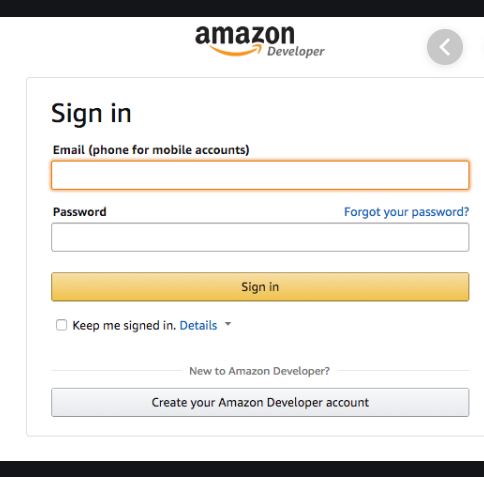**Caption:**

The image displays the Amazon Developer sign-in page, bordered at the top and bottom by black horizontal strips. The main background is white. Centrally positioned is the Amazon logo with the word "developer" directly below it in gray font. A gray circle containing a white left arrow is situated to the right of the logo.

Beneath this, there is a partially cut-off sign-in box with a light gray outline. Inside the box, the following elements are sequentially arranged:

1. The text "Sign-In" in bold black font.
2. The labels "Email," "Phone," and "Phone or mobile accounts" in black above an orange-outlined data field.
3. The label "Password" followed by the clickable text "Forgot your password?" in blue, and a data field outlined in gray.
4. A yellow "Sign-In" button with black text, matching the width of the data fields.
5. The option "Keep me signed in" with a drop-down "Details" link in blue, and an unchecked checkbox.

No information has been entered into any data fields.

Towards the bottom, the text "New to Amazon Developer?" is enclosed by horizontal gray lines, rendered in gray font. Below it is a gray button with the text "Create your Amazon Developer account" in black font.